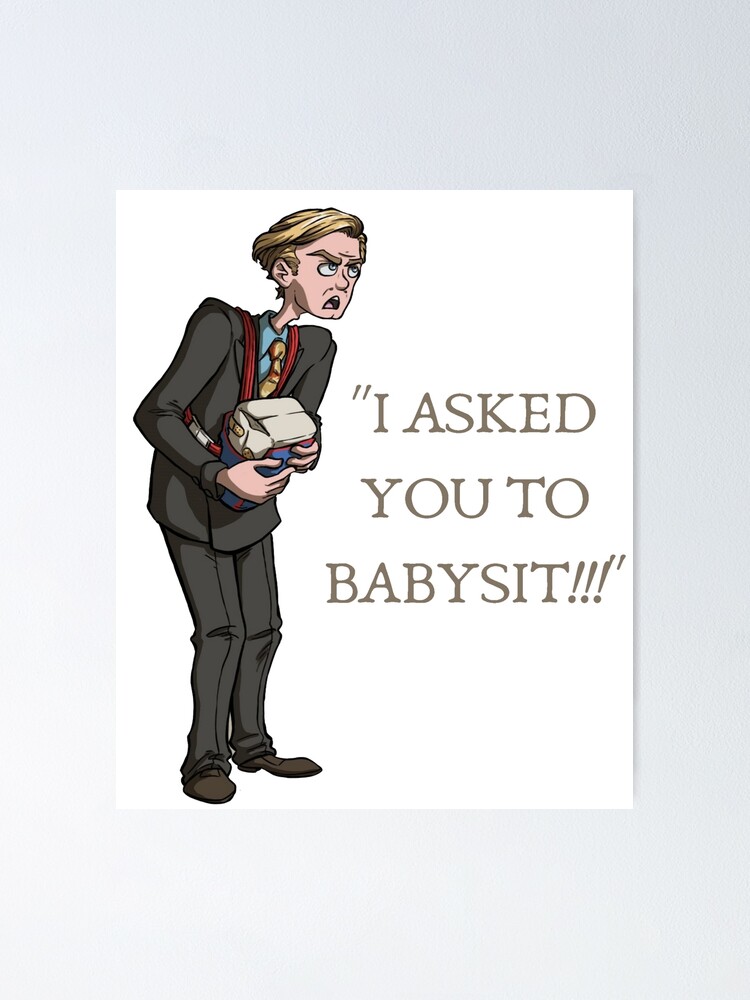The image depicts an animated drawing of a visibly annoyed man with blonde hair and pale skin, wearing a gray suit, blue collared shirt, and an orange (or possibly darker yellow) tie. He has brown shoes, and his exaggeratedly large feet add a humorous touch to his otherwise stern demeanor. His heavy eyebrows are furrowed over his light-colored eyes, and his mouth is open in a frown as if he is speaking angrily. The man is holding a bag of flour close to his chest, and there is also an unidentifiable object next to it. He stands against a very light gray to white background. To the right of him, in large brown letters and inside quotation marks, is the exclamation "I asked you to babysit!!!". This drawing is presented on a white piece of paper.